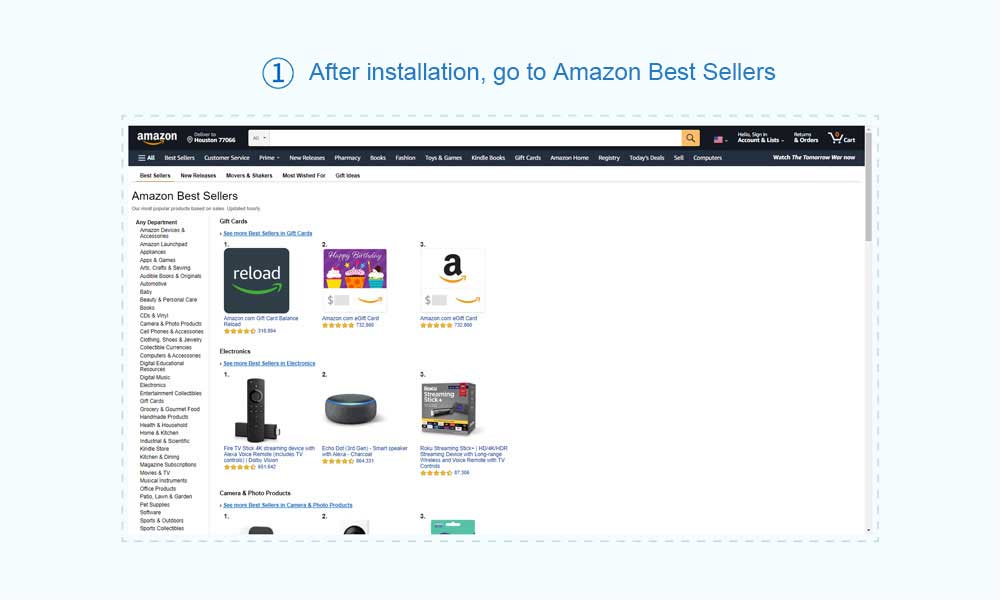The image features a baby blue background with an inset depicting the Amazon website. This inset image, outlined with small dash lines resembling a cut-out or a sticker, appears to have been manipulated in a paint program. At the top center of the image, the text "1. After installation, go to Amazon Best Sellers" is displayed in blue font, suggesting a step-by-step guide.

The inset showcases the Amazon Best Sellers page, where multiple categories such as Gift Cards, Electronics, and Camera & Photo are clearly visible. The left side of the page displays a comprehensive list of Amazon departments. Across the top navigation bar, numerous categories, including Customer Service, Pharmacy, Socks, Fashion, and Toys & Games, are outlined. The Amazon interface features familiar elements such as an empty cart icon, a sign-in button, and a prominent white search bar at the top.

Overall, the image appears to provide instructional guidance for users, directing them on how to navigate to the Amazon Best Sellers page after completing an installation process.